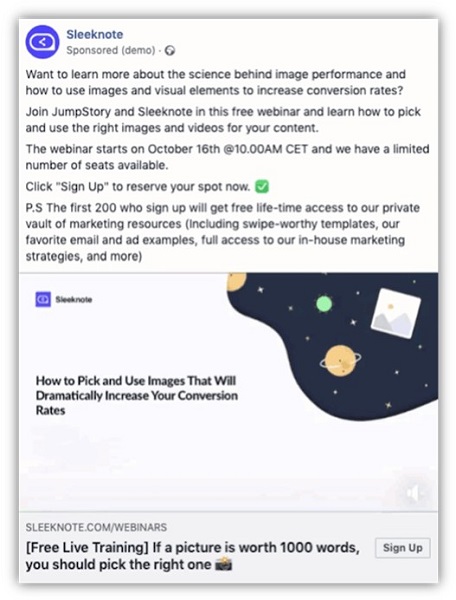The background of the image features a predominantly white upper section. In the left-hand corner, there is a purplish circle containing a white oval outline. An arrowhead, pointing towards the left and colored in white, is also present within this circle. The word "Sleep Note" is displayed in purple text, followed by "sponsor" in black text with "demo" in parentheses. 

An invitation message follows, encouraging users to join Drum Story and Sleep Notes for a free webinar that covers the science behind image performance, as well as the use of visual elements to increase conversion rates. The webinar is scheduled to start on October 16th at 7:10 a.m. CET, and attendees are invited to reserve their spots due to limited availability. 

A call-to-action button featuring a green box with a white checkmark is included. An additional note (P.S.) mentions that the first 200 sign-ups will receive free lifetime access to a private vault of marketing resources, which includes swipe-worthy templates, favorite email and ad examples, full access to in-house marketing strategies, and more.

A horizontal purple box with a white oval stating "Sleep Notes" contains a black text line that reads, "How to pick and use images that will dramatically increase your conversion rates."

In the right-hand corner, the background transitions into an animated outer space theme, featuring black and white stars, along with what appears to be an orange ringed Saturn. The bottom of the image is accented by a thin gray line.